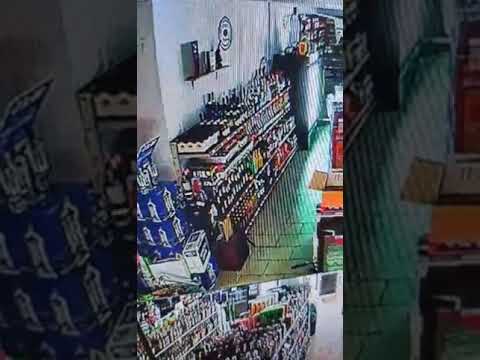The image appears to be a still from a grainy, pixelated color surveillance camera inside a convenience store. The scene mainly focuses on shelving units along the left wall, filled with liquor bottles and cases of other items, possibly beer or soft drinks, stacked on the floor at the end of the aisle. The lower section of the image features a partially visible frame showing a different part of the store, with additional nondescript shelves further in the background. The scene is captured during daylight hours, and the store appears empty, without any customers present. The floor is tiled, and there are various decor items hanging on the walls. The image includes a palette of colors such as blue, white, green, red, orange, purple, and tan, and there is no visible text anywhere within the frame.